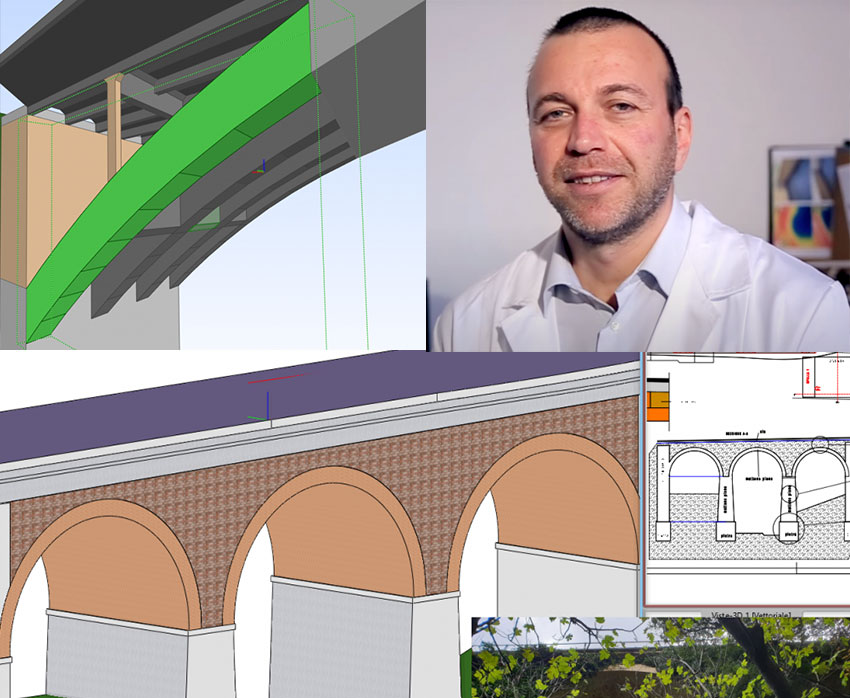The image is a detailed and organized collage that highlights an architectural design process. It is divided into several distinct sections. In the top right, there is a photograph of a smiling Black man with a slight beard and short haircut, dressed in a white lab coat over a light blue or white shirt, suggesting a professional or academic setting. Behind him is a blue and orange painting in a black frame. To the left of his photograph is a detailed colored drawing of a bridge with a green arch and several supporting gray arches below it. Beneath this drawing is another depiction of the bridge, illustrating its structural components with cylindrical openings and a purple roof, which may serve as an underpass for boats. Adjacent to this, on the lower right, is a black and white schematic of the same bridge, capturing the intricate details of its design. In the bottom right corner is a small, thin rectangular image showcasing a tree with leaves, possibly indicating a natural element related to the architectural plans. This collage reflects different phases and perspectives of the bridge's planning and design process, presumably curated by the man in the photograph.